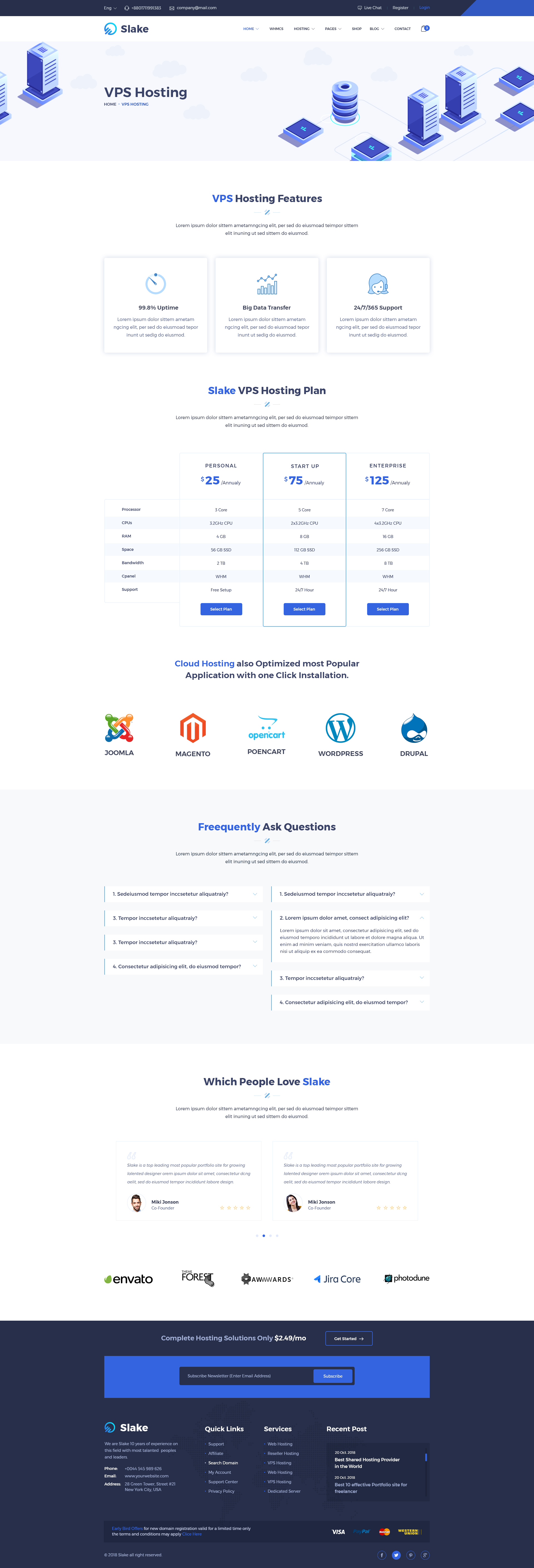The website for the brand Slate features a prominent banner at the top of the homepage, showcasing their VPS hosting services. The banner is visually engaging, displaying various graphical representations of virtual machines and servers. Directly beneath the banner, the phrase "VPS Hosting Features" is prominently displayed, though some text is small and difficult to read. The site's primary colors are a blend of bluish purple and white, offering a clean and modern aesthetic.

The webpage is extensive, outlining numerous features of their VPS hosting services in detail. The pricing section is clearly defined, with three columns indicating different plans: $25, $75, and $125. Beneath these pricing columns, small logos add an extra layer of information and branding.

Continuing down the page, a small rectangular box is dedicated to frequently asked questions (FAQs), providing users with common inquiries and their answers. Following the FAQ section, there's a segment titled "Which People Love Slate," featuring headshots and testimonials from two satisfied customers.

At the very bottom of the page, a set of links guides users to various sections of the website. The word "Slate" is repeated, emphasizing brand identity, and users can navigate through different categories to explore more features or information relevant to their needs.